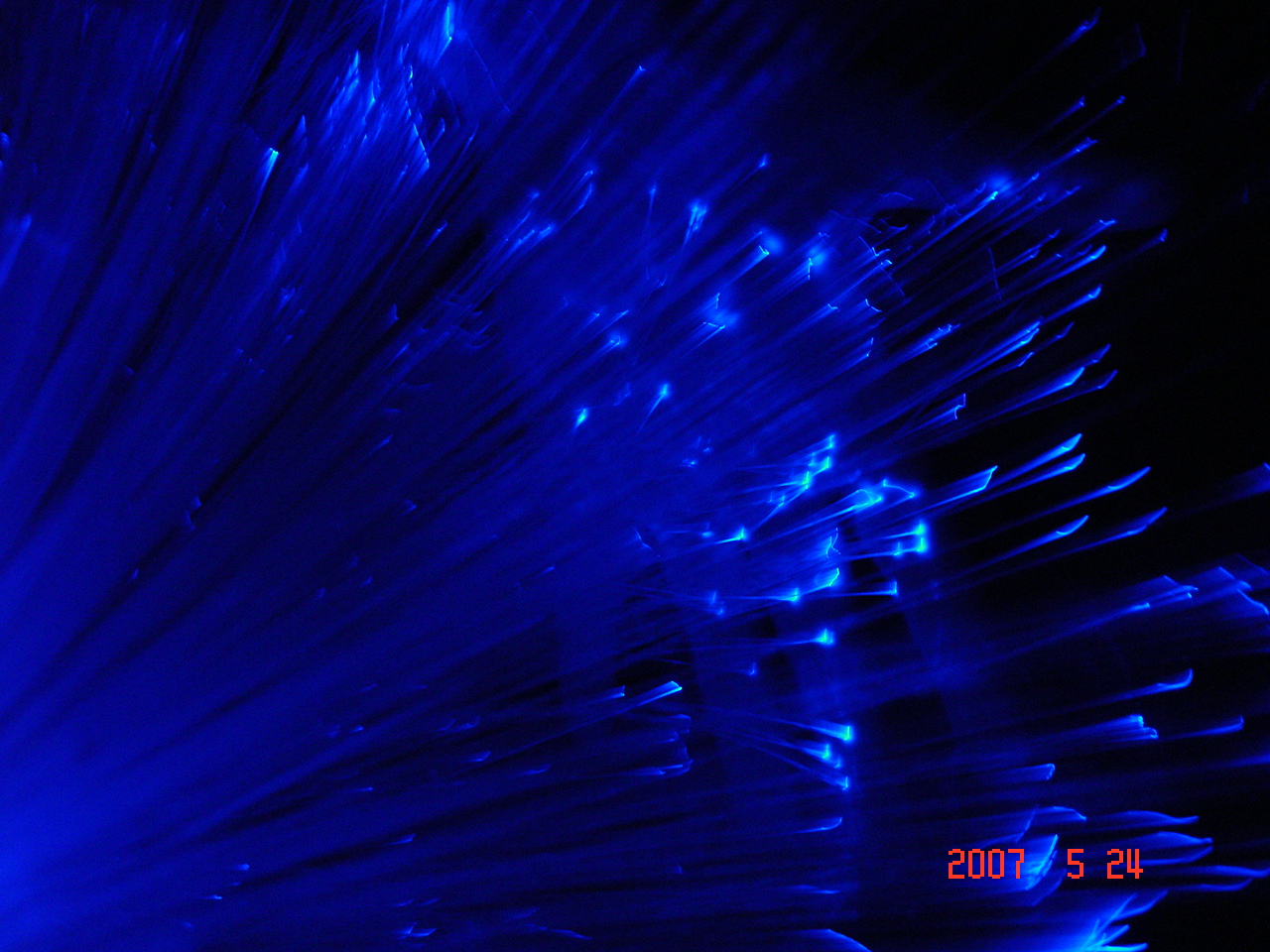In this visually captivating image, a rectangular photograph slightly wider than it is tall, we are greeted by a dark blue, nearly black background. Sweeping across the frame from the lower left corner to the upper right are hundreds of fiber optic strands, brilliantly illuminated at their tips. These glowing fibers, evoking a sense of motion as if they are gently waving or squiggling, give the impression of an ethereal light show or an underwater scene.

The brilliant blue of the fibers dominates the lower left portion of the image, gradually merging with the black background as they extend upwards and to the right. These delicate strands create a mesmerizing pattern, resembling an intricate piece of artwork. Amongst the vibrant blue, there appears to be a ghostly, translucent image that some might liken to an octopus with its tentacles trailing behind it.

In the lower right corner, the date "2007 5 24" is prominently displayed in digital red print, adding a temporal context to this abstract and fluid composition.